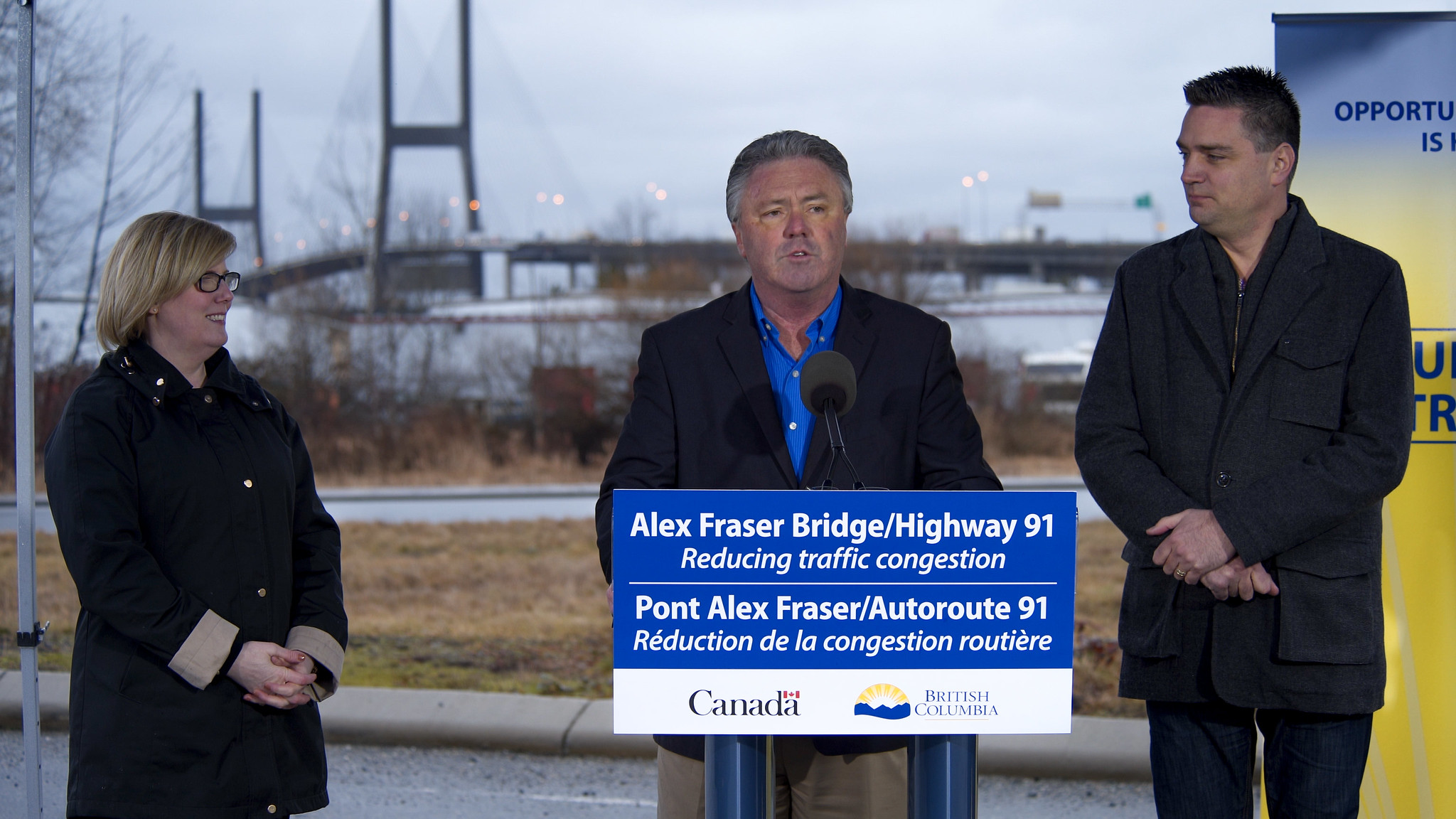This photograph captures an outdoor event featuring a podium centrally placed with a poster that reads, "Alex Fraser Bridge / Highway 91, Reducing Traffic Congestion, Pont Alex Fraser / Autoroute 91, Reduction de la Congestion Routier, Canada, British Columbia." A man stands behind the podium, speaking into a microphone. He is dressed in a blue shirt and a black coat. Flanking him are two individuals: to his left stands a woman in a black coat and glasses, attentively watching him, and to his right stands another man also in a black coat and black pants, similarly focused on the speaker. The backdrop reveals a scenic setting with a large bridge spanning over water, a stretch of roadway, dry grassy ground, and an expansive sky, indicating a waterfront location. This appears to be a formal announcement or speech, likely by a political figure discussing infrastructure improvements.